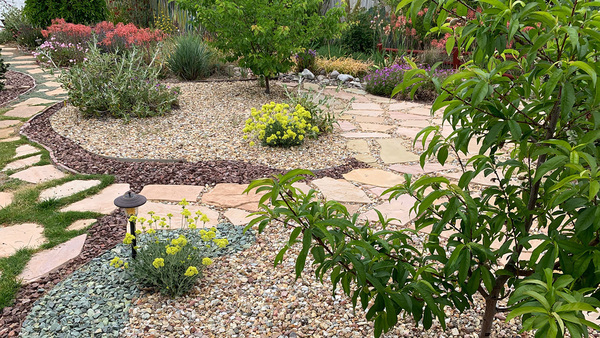The photograph depicts a lush landscape garden, possibly a backyard, featuring a winding stone pathway that meanders through various sections of the garden. The ground is adorned with intricate designs made from pebbles and flat stones of different sizes and shapes. Several circular stone walkways are present, each encircling distinct plant arrangements. One such circle contains three bushes and a small tree, while similar flora populate another adjacent circular pattern. The garden bursts with color from patches of purple, yellow, and pinkish-red flowers, in addition to diverse shrubs and smaller plants. The scene showcases a variety of landscaping rocks in brick, gray, and tan hues, adding to the decorative appeal. Lavender bushes and other flowering plants provide a vibrant backdrop, with green leaves abundant throughout. A large green tree dominates the foreground, and the sky above is hazy and cloud-covered, suggesting a midday setting with diffuse lighting and no distinct shadows.